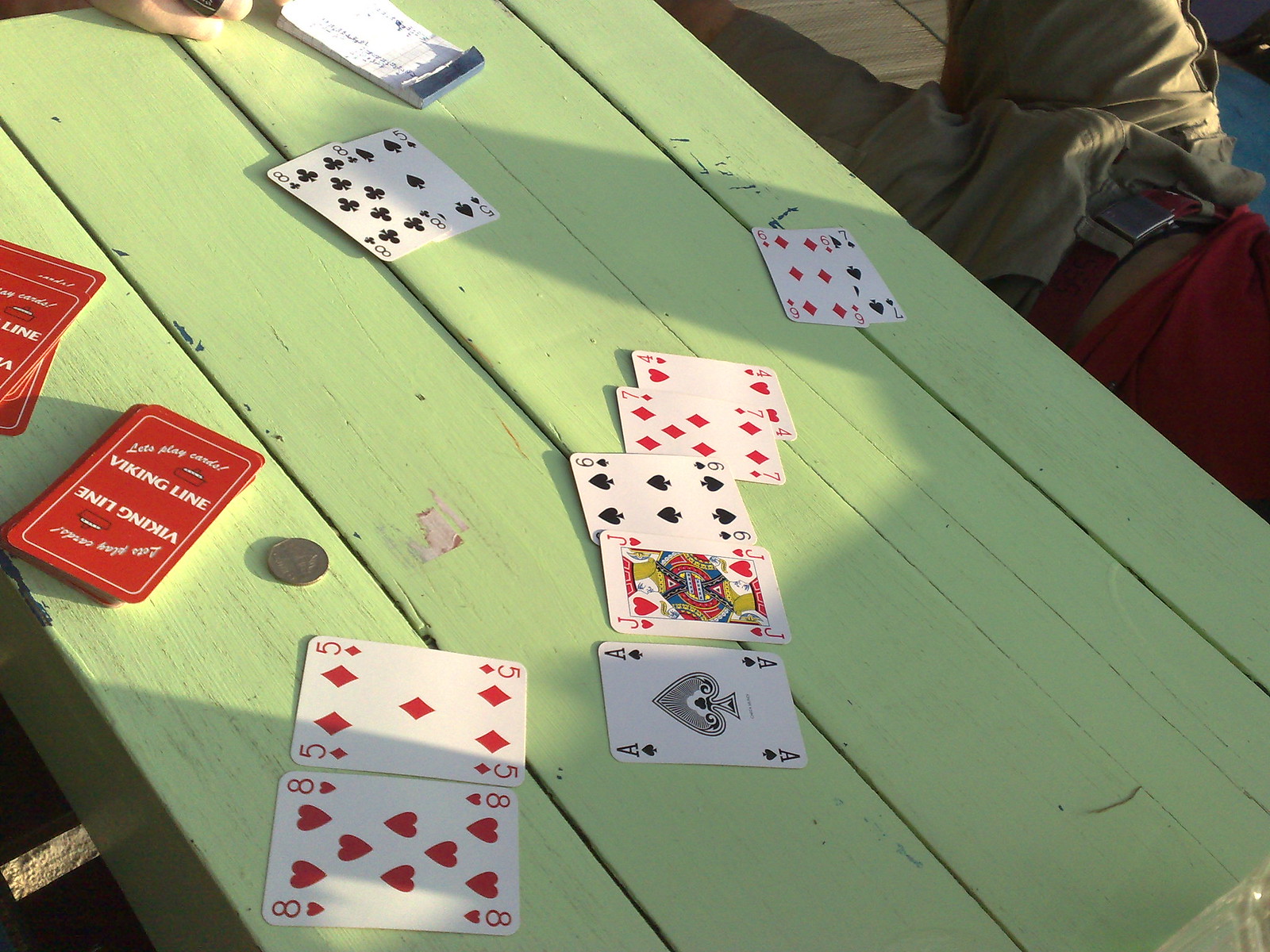This outdoor scene features a classic picnic-style table painted in a refreshing mint green hue. Spread across the table's surface is a collection of playing cards arranged in various formations. On the left side, two red cards, the five of diamonds and the eight of hearts, are situated next to each other. Adjacent to them lies a sequence of five cards neatly aligned: the black ace of spades, the red jack of hearts, the six of spades, the seven of diamonds, and the four of hearts. 

Moving further along, another duo of cards appears—the red six of diamonds and the black seven of spades—resting side by side. Nearby, the black eight of clubs and the five of diamonds are placed together. Adding to this tableau, a separate pile of cards sits flipped over on the opposite side of the table, revealing the card back, which displays "Viking Line" on a red background with the phrase "Let's Play Cards" elegantly written in white cursive.

The scene is sunlit, casting a distinct shadow across the table. Beside the table, a male figure reclines on the bench, dressed in khaki pants with a red belt featuring a silver buckle and wearing a red shirt. This detailed arrangement creates a serene, inviting atmosphere ideal for leisurely outdoor gaming.